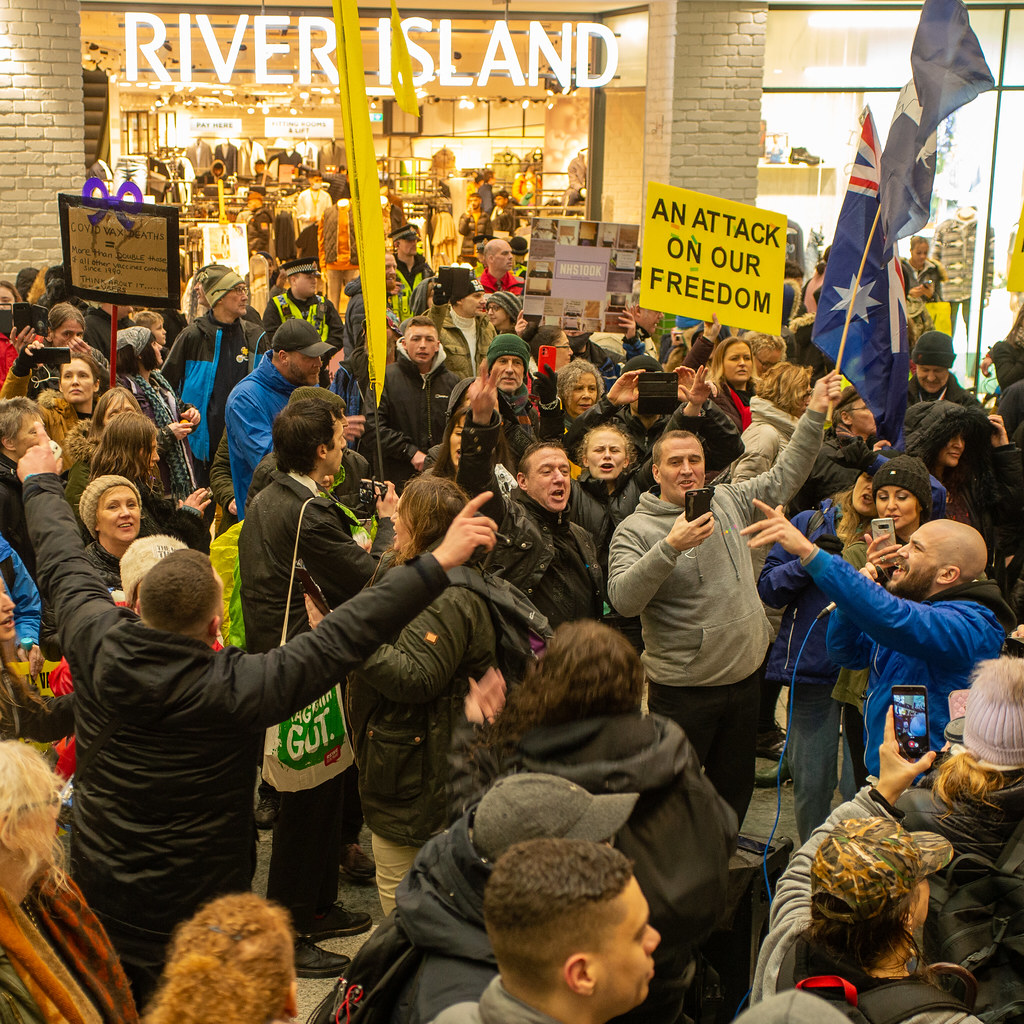In this photograph, a large group of people are gathered outside a River Island store, which is prominently marked by bright white, all-capital letters in the upper left corner of the image. The crowd appears to be participating in a demonstration, with many individuals holding signs, flags, and megaphones. A striking yellow sign stands out with the bold black text, "An Attack on Our Freedom." The flags being waved include a notable dark blue one featuring a silver star, although another blue flag is partly obscured. Most of the demonstrators are dressed in coats and hats, suggesting it is a chilly, possibly autumn or winter day. Among the crowd, some people have their cell phones out, capturing the event. The person positioned in the lower right corner is distinctively wearing a baseball cap.